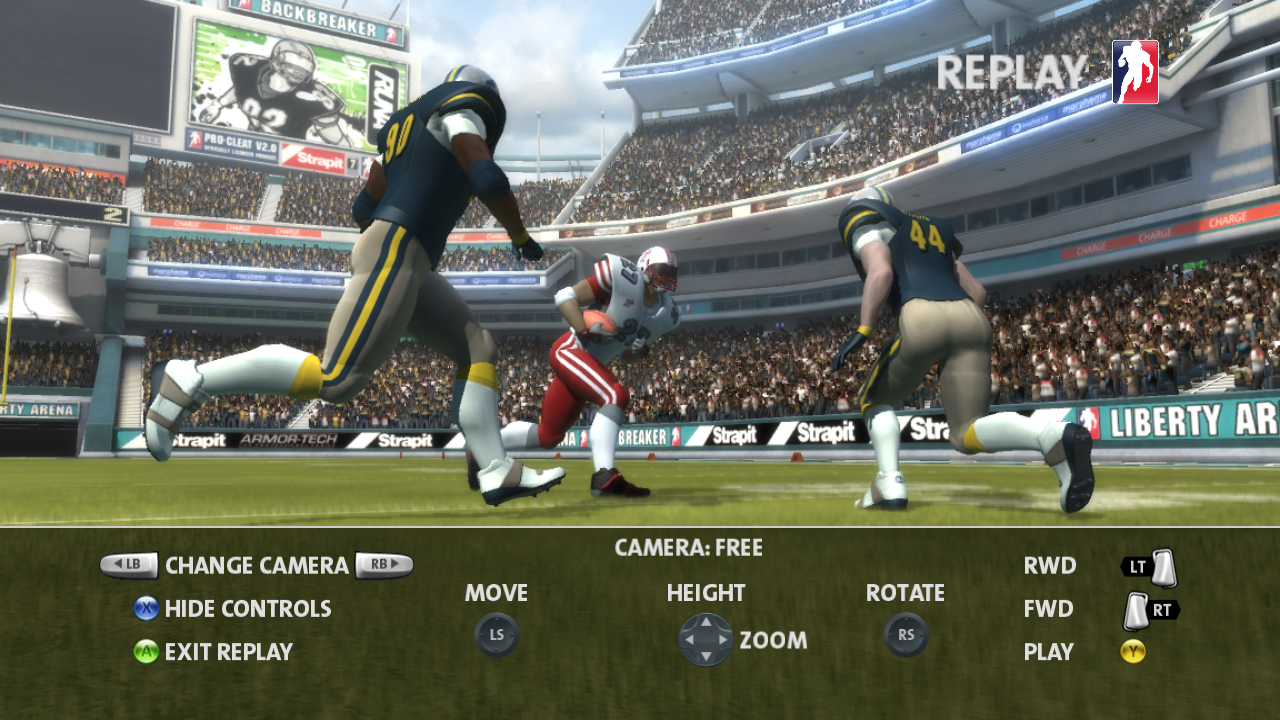This image is a screenshot from the football video game Madden, featuring an in-game replay mode. The scene captures three football players in dynamic motion on a green grass field. Two players, wearing black jerseys with yellow accents, likely from the Pittsburgh Steelers, are positioned on the left and right sides of the screen. The left player is number 90 and the right player is number 44, both sporting navy-colored jerseys with gray pants, detailed with yellow stripes. The central player, in a gray and red uniform, possibly representing the Kansas City Chiefs, appears to be engaged in a struggle for the football with the player on the right.

In the background, a packed stadium sets the stage, complete with a jumbotron in the upper left corner displaying a close-up of player number 22, clad in a dark uniform. A Philadelphia Liberty Bell replica is prominently featured on the left side of the stadium. The top right corner of the screen is marked with the word "REPLAY" alongside the NFL logo. The bottom strip of the image shows various game controls and settings such as "change camera," "hide controls," "exit replay," "move camera," "free rotate," "RWD," "FWD," and "play."